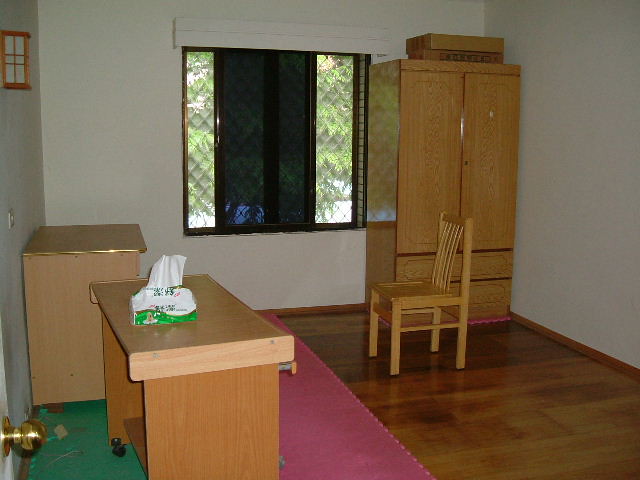This indoor photograph captures a cozy, small room painted in white with brown wood molding along the floor. Dominating the far wall is a large, rectangular window, revealing a vista of trees and greenery outside. To the right of the window stands a tall, honey oak-colored dresser, slightly extending in front of the window, accompanied by a wooden chair oriented to the left. The floor is a polished hardwood, accentuated by two colorful mats: a bright green mat beneath a pair of brown desks on the left side of the room, with a pink mat in front of them. The two desks differ slightly in design—one is stationary with a box of tissues atop it, while the other, possibly on casters, appears mobile and versatile. A subtle light fixture is mounted on the wall above the desks. In the bottom right corner, a glimpse of a door with a golden doorknob adds to the room's charm. The consistent honey oak finish across the furniture pieces ties the space together harmoniously.